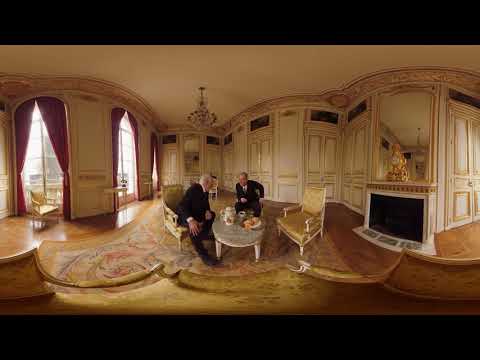This image depicts a grand, ornately decorated reception room often found in stately homes or government buildings. The room features high, eggshell-colored walls contrasting with a slightly darker white ceiling, from which a chandelier hangs, unlit due to the daytime setting. On the left, tall windows stretch from floor to ceiling, adorned with heavy burgundy curtains held back by ties. 

In the center of the room, against an opulent backdrop, are two men seated in vibrant yellow chairs around a low, white coffee table. Both men, who are elderly and dressed in black suits with white shirts, appear engaged in deep conversation. The man on the left has graying hair or is possibly balding, facing right toward the other gentleman. His counterpart is seated facing left at a three-quarter angle, adding to the sense of interaction between them. On the table, a teapot is accompanied by an assortment of snacks or biscuits, suggesting a casual yet refined meeting.

To the right of the second man, an empty chair awaits, matching the ornate, yellow padded style seen throughout the room. The wooden floor is partially covered by throw rugs that blend yellow and brown hues with touches of red. On the far right, a white fireplace with a red brick trim takes a prominent position, crowned by a tall painting. The room's back wall features scalloped, ornate panels, indicating intricate architectural detailing, while the space beyond the fireplace appears to open into another area, possibly a hallway. This elegant setting evokes a sense of regality and formal discourse.